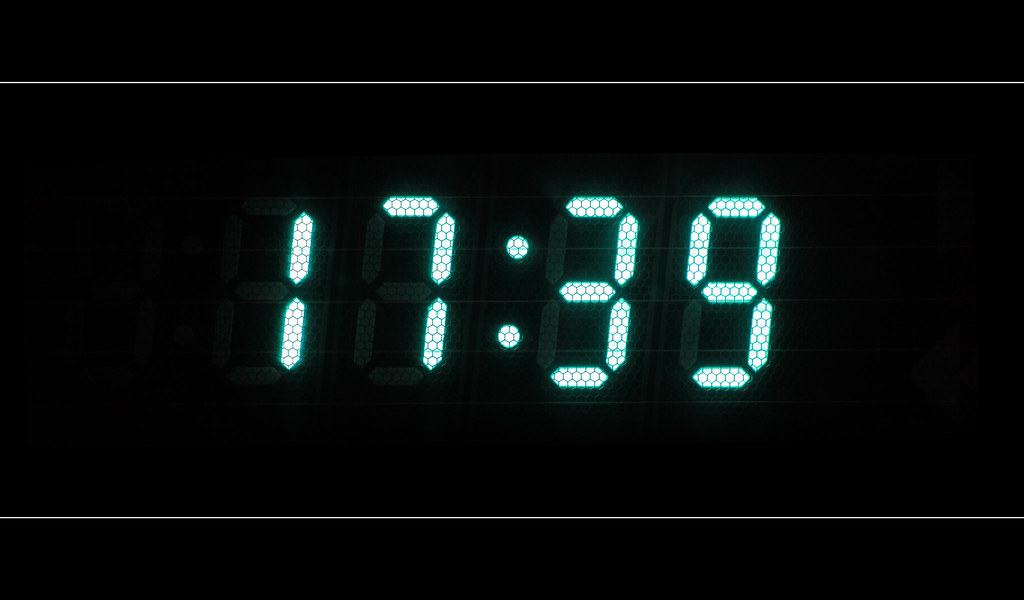This is a close-up color photograph of a digital clock face displaying the time 17:39 on a 24-hour scale. The numbers are a vibrant, almost neon, mint green color and are highly detailed, down to the individual pixels, which have a floral-like black pattern. All other elements are set against a dark, black background that highlights the light-emitting digits. At both the top and bottom of the image, there is a thin, white stripe running horizontally. The numbers, "17:39," are prominently centered between these lines. Additionally, there is a faint, ghosted imprint of other numbers visible, adding an intriguing layer to the image's close-up perspective. No other objects are present in the scene, suggesting the photo may be of a digital timer on a microwave or an oven.